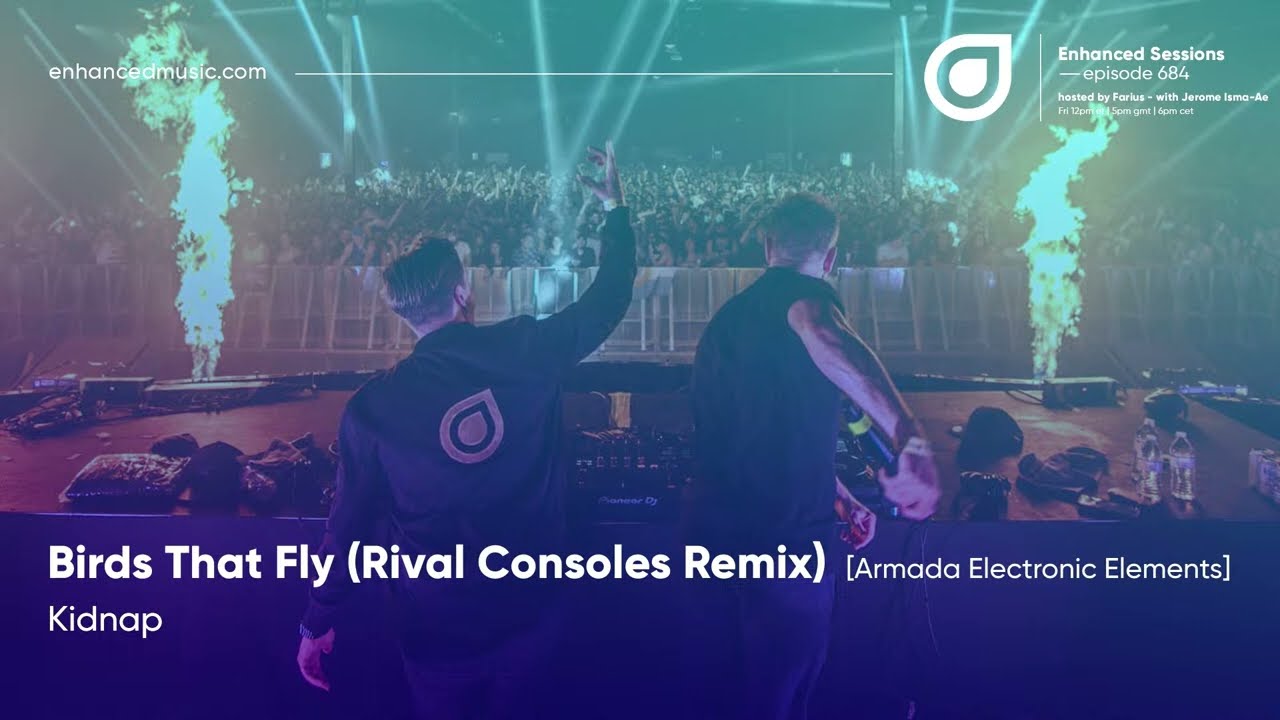The image depicts a high-energy concert setting featuring two men on a stage, likely DJs, who are central to the scene. Their backs are turned to the camera as they stand in front of a music console or podium. Both performers are dressed in black. The atmosphere is vibrant with green spotlights illuminating the air, and there are dramatic flames shooting up from flat brown tubes on either side of the stage. A large crowd is visible behind the stage, separated by a fence. The bottom of the image features text in white font that reads, “Birds That Fly, Rival Consoles Remix, Armada Electronic Elements, Kidnap.” Additional text such as "Enhanced Sessions Episode 684 hosted by Far Less with Jerome Isma I Friday 12 p.m. and 5 p.m. GMT 6 p.m. CET" and "enhancedmusic.com" are positioned at the top corners, providing more details about the event. The entire scene is enveloped in fog or smoke, adding to the dramatic and electrifying ambiance.